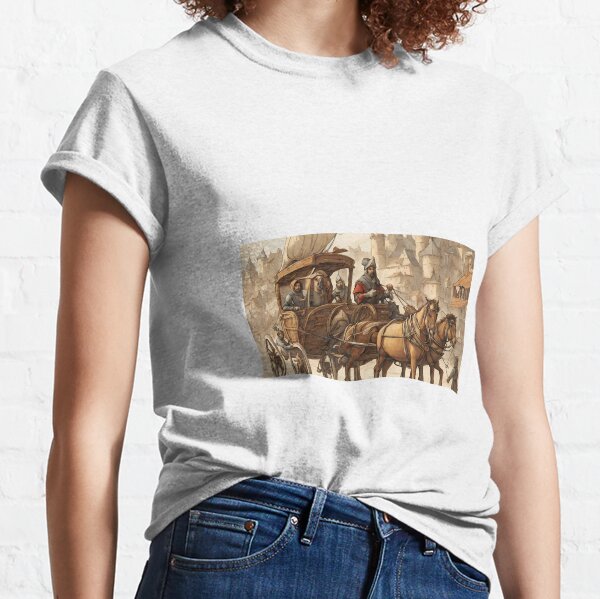This photograph captures a woman with curly red hair, likely Caucasian, wearing a white t-shirt with short, cuffed sleeves, partially tucked into her bright blue jeans. The focal point of the image is the detailed print on the t-shirt, depicting an old-time scene of a horse-drawn carriage with two horses, a driver with red sleeves, and passengers in the cart, set against a backdrop of medieval-style buildings. The print is in a rectangular, landscape orientation, primarily in orange and grey tones. The overall setting appears to present the woman modeling the t-shirt, as the crop of the image frames her from the neck to the waist, with the background being a plain white color. The interplay of shadow around the neckline and the angle of the shot suggests a natural, casual pose, emphasizing the design and fit of the shirt.